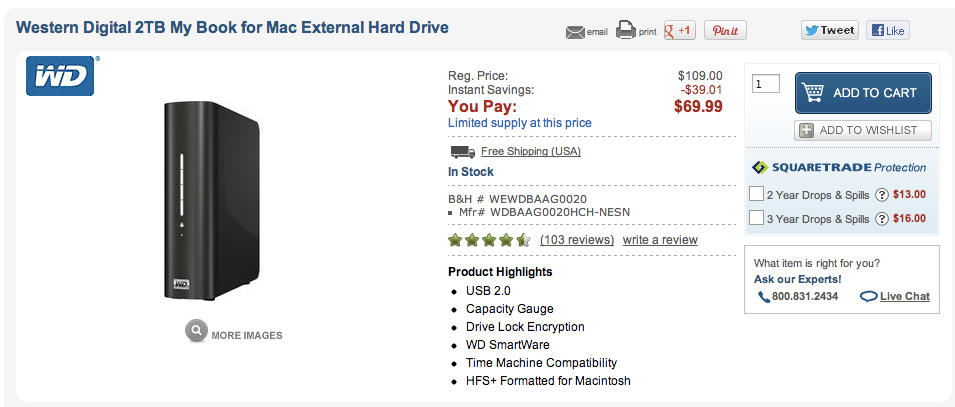In this image, there is a listing for a Western Digital 2TB My Book for Mac external hard drive. The drive is sleek and black, featuring the Western Digital logo prominently at the top left. The pricing details indicate a regular price of $109, with an instant savings of $9.01, reducing the final cost to $69.99. Shipping is free within the USA. The product is currently in stock and offers several notable features: USB 2.0 connectivity, a capacity gauge, drive lock encryption, WD SmartWare software, Time Machine compatibility, and HFS+ formatting for Macintosh systems. Additional options include R2Cards and an R2 wishlist, as well as SquareTrade protection plans: a 2-year drops and spills coverage for $13 and a 3-year plan for $16. For personalized assistance, the listing also offers the option to ask product experts or engage in a live chat.